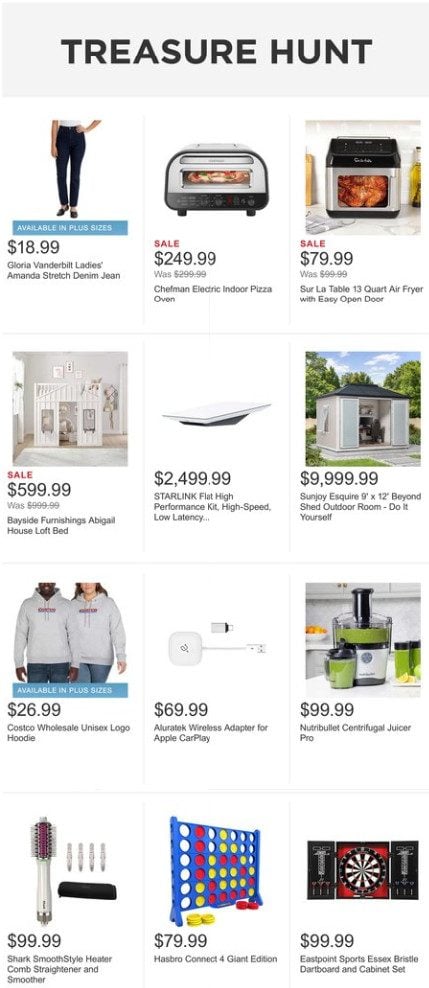Here is a detailed and clean caption:

---

This image is a screenshot of a web page showcasing a variety of items available for purchase. At the top, in a mid-gray rectangular box with bold black text centered, it reads "Treasure Hunt".

- **Left Hand Side**:
  - **Leggings**:
    - A pair of black leggings is displayed on a Caucasian woman wearing a tight-fitting white shirt and brown shoes.
    - Below, in a blue rectangle, it states "AVAILABLE IN PLUS SIZES" in all caps white text against a mid-blue background.
    - Price: **$18.99** in black.
    - Description: **Gloria Vanderbilt Ladies Amanda Stretch Denim Jeans**.
  - **Toaster Oven**:
    - A toaster oven resembling a Ninja Foodi is shown with a silver top and black bottom.
    - "SALE" is written in red, followed by **$249** in black.
    - Original price: **$299.99** with a line through it.
    - Description: **Chefman Electric Indoor Pizza Oven**.
  - **Air Fryer**:
    - A silver air fryer with a black top and bottom is displayed on a white and gray marble countertop against a white wall, with a tan cabinet to the left.
    - "SALE" in red, followed by **$79.99** in black.
    - Original price: **$99.99** in gray.
    - Description: **Sur La Table 13 Quart Air Fryer with Easy Open Door**.

- **Center Segment**:
  - **Furniture**:
    - A white piece of furniture, appearing as a house loft bed with a mirror.
    - "SALE" in red: **$599.99** in black.
    - Original price: **$999.99** with a line through it.
    - Description: **Bayside Furnishings Abigail House Loft Bed**.
  - **Table**:
    - A white table with a black base.
    - Price: **$2,499.99** in black.
    - Description: **Starlink Flat High Performance Kit, High Speed Low Battery ...**.
  - **Shed**:
    - A silver shed with a dark blue roof, surrounded by dark gray items and shown on a concrete path with dark green trees and a blue sky with white clouds.
    - Price: **$9,999.99** in black.
    - Description: **Sunjoy Esquire 9' x 12' Beyond Shed Outdoor Room-Do It Yourself**.
  - **Hoodies**:
    - Two individuals in gray sweatshirts with red writing. The first is an African American male wearing dark blue jeans; the second is a Caucasian female with long brown hair wearing light blue jeans.
    - Below, in a mid-blue rectangle with all caps white text: "AVAILABLE IN PLUS SIZES".
    - Price: **$26.99** in bold black.
    - Description: **Costco Wholesale Unisex Logo Hoodie**.

- **Right Hand Side**:
  - **Charge Cable**:
    - A light gray and white charge cable.
    - Price: **$69.99** in black.
    - Description: **Allotech Wireless Adapter for Apple CarPlay**.
  - **Juicer**:
    - A black and dark green blender or food processor with white cabinets in the background.
    - Price: **$99.99** in black.
    - Description: **Nutribullet Centrifugal Juicer Pro**.
  - **Curling Iron**:
    - A white and silver curling iron with purple and hot pink accents, alongside accessories and a black holding case.
    - Price: **$99.99** in black.
    - Description: **Shark Smooth Style Heater Comb Straightener and Smoother**.
  - **Connect 4**:
    - A dark blue Connect 4 game with dark red and bold yellow chips.
    - Price: **$79.99** in black.
    - Description: **Hasbro Connect 4 Giant Edition**.
  - **Dartboard**:
    - A dartboard set with a red background, circular black board with silver portions, black and white bands on the interior, red lining, and black sections for holding darts and other items (too small to be seen clearly).
    - Price: **$99.99** in black.
    - Description: **East Point Sports Essex Bristle Dartboard and Cabinet Set**.

---